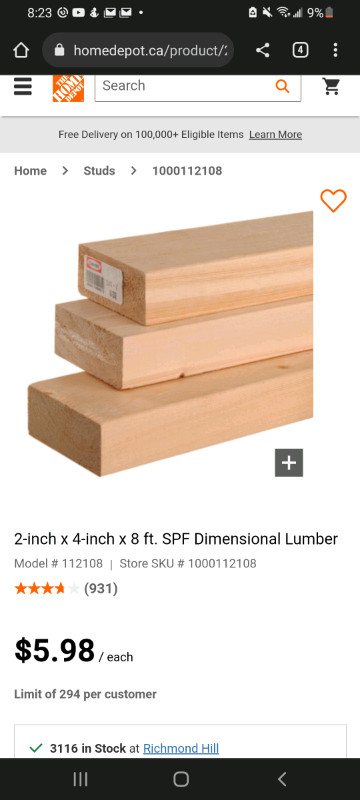A detailed caption for the image could be formulated as follows:

"The image displays the Home Depot website as viewed on a smartphone. The top section of the screen features the status bar with several icons and indicators. On the upper left, the number '823' is displayed alongside a YouTube icon, possibly some mail icons, and on the right, indicators for 'No Sound', Wi-Fi signal, cell signal, and a '9%' battery status, which is shown in red.

Below the status bar, the webpage header includes a navigation bar with various icons: starting from the left, there is a home icon, a search field that shows 'homedepot.ca/products/', followed by a share icon represented by four squares in a larger square pattern, and three vertically aligned dots, all set against a black background with white font.

On the bottom section of the screen, a white background hosts further navigation options. On the left, there are three horizontal lines stacked to indicate a menu. Next to it is the Home Depot logo, an orange square with the words 'Home Depot' written in white. Adjacent to the logo is a search bar with the placeholder text 'search' in gray, accompanied by a magnifying glass icon that is green and orange. Further to the right, there’s a black shopping cart icon.

Below these elements, a banner announces, 'Free delivery on 100,000+ eligible items', with a 'Learn More' link. Beneath this, navigation breadcrumbs read, 'Home > Studs > 1000112108', indicating the user's path through the site. The main content features an image of three neatly stacked 2x4 lumber pieces.

The distinct sections and visible elements provide a comprehensive view of the Home Depot mobile website, capturing both functional icons and navigational cues."